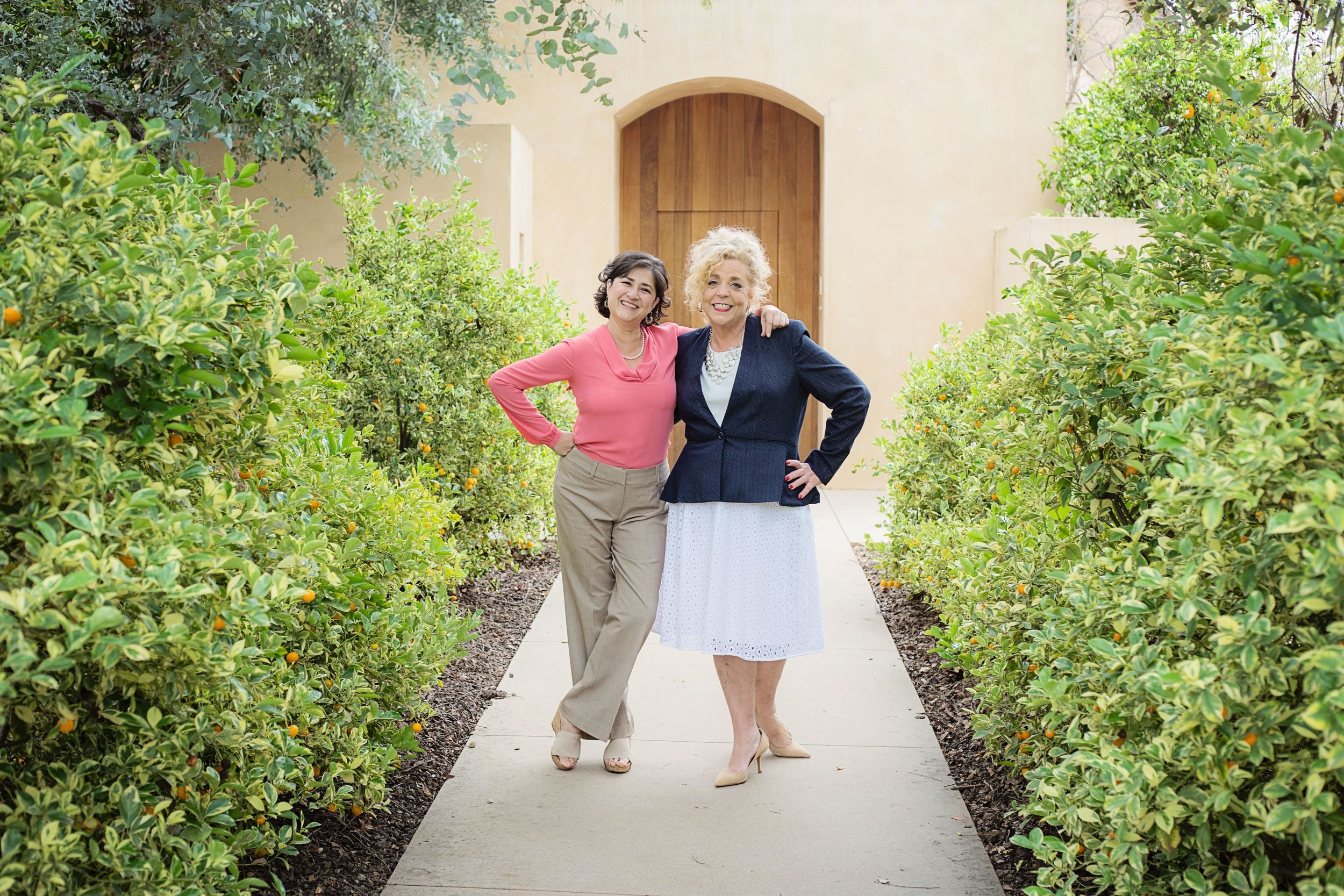The photograph captures a color image of two women, standing on a paved pathway flanked by lush green shrubs. The pathway leads to a grand wooden door set into a beige stucco building, possibly part of a church or a similar complex. Both women are standing close together, with their arms wrapped around each other's backs and shoulders, radiating happiness with their big smiles. 

The woman on the left, who appears to be around 50 years old, has brown hair, and is dressed in a pink long-sleeve top paired with light khaki pants and sandals. She stands with her legs crossed and her right elbow bent, her hand resting on her hip, tilting her head slightly toward her companion. The woman on the right, approximately 55 years old, sports fuzzy blonde hair styled atop her head. She is dressed in a navy blue jacket over a white, full-skirted dress, and wears high heels. She mirrors the pose of the first woman, with her left elbow bent and her hand on her hip, while the other woman's hand rests on her shoulder. The shrubbery surrounding them features small, possibly orange or yellow, fruits.

The overall atmosphere of the image conveys a sense of joy and togetherness, capturing a candid moment between the two women against a picturesque and serene backdrop.